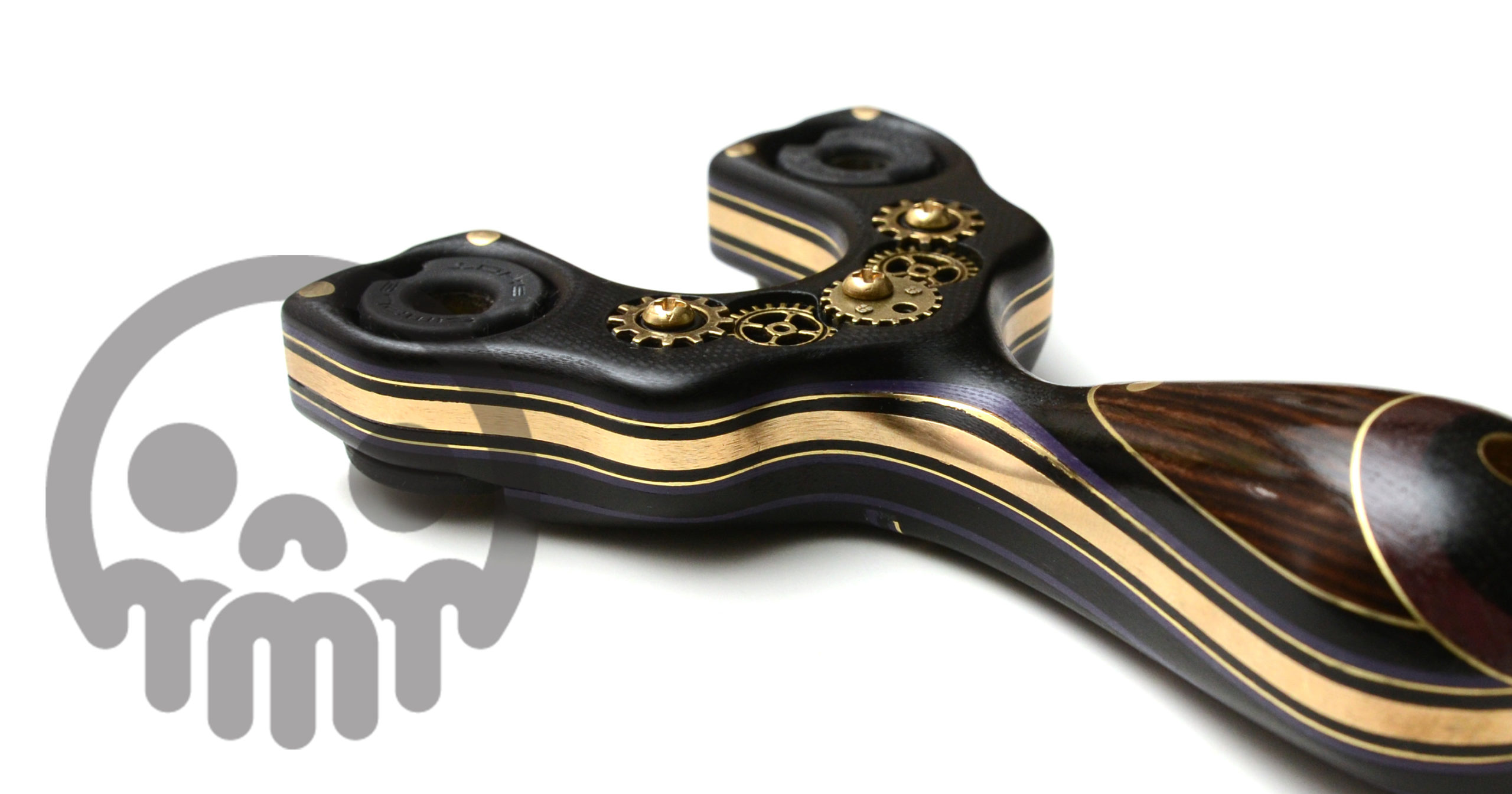This image showcases a meticulously crafted, ornate slingshot-shaped object, though it lacks the traditional elastic band for slinging. The piece features a short, rounded handle made of high-quality wood, with a black finish accented by a gold stripe running along its edge and hints of brown in the handle's coloration. At the top section, which resembles the arms of a Y-shape or wishbone, there are multiple gold gears—specifically five—adding to its intricate design. Positioned to the left of this device is a gray stamped image of a face, resembling a stylized skull with circular eyes, an upside-down U for a nose, and a mouth area that includes a series of M-like humps. The overall craftsmanship and detailed elements suggest this could be more than a simple tool, maybe even an artistic piece or a conceptual design.